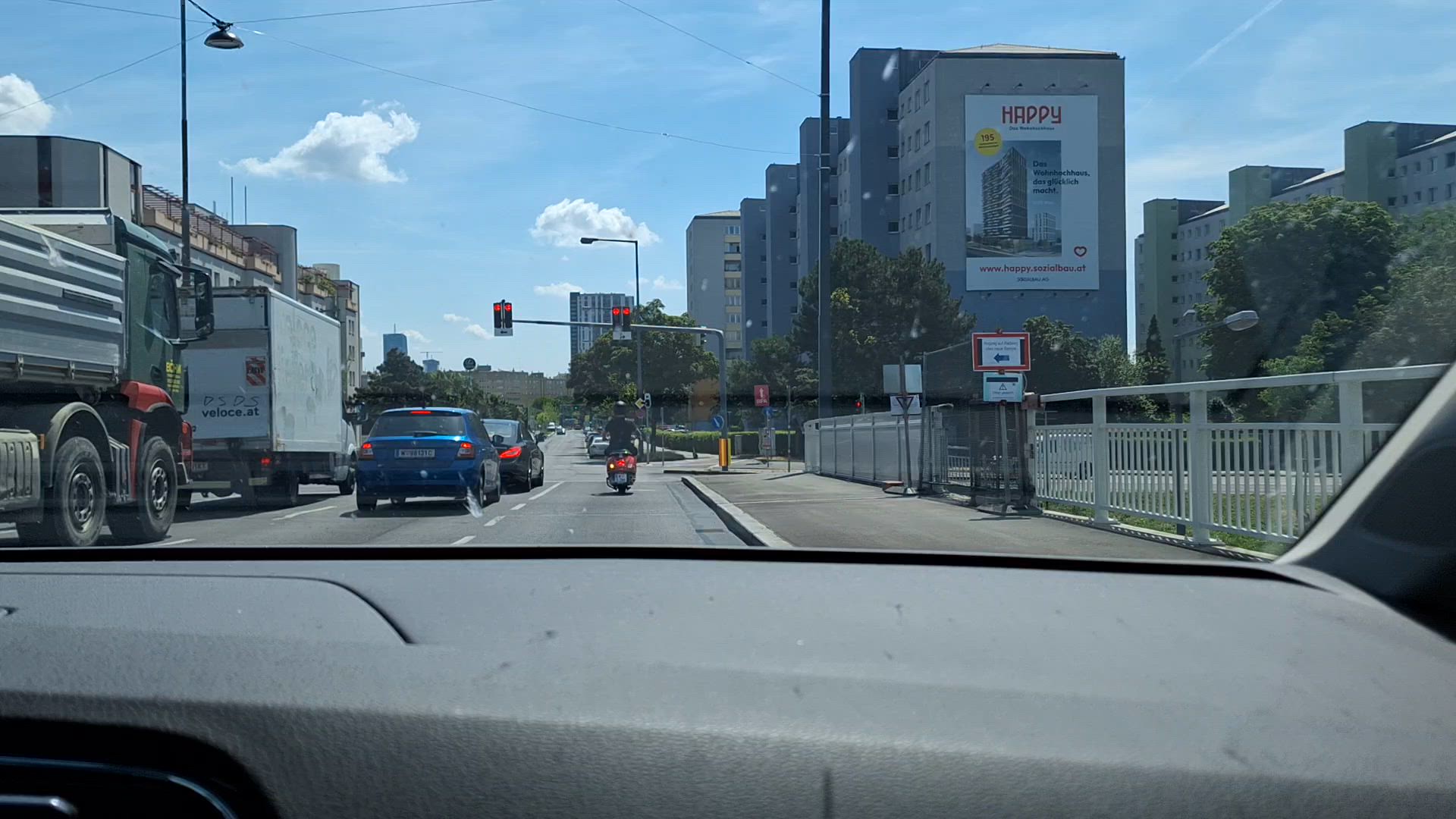This detailed outdoor photograph captures a bustling cityscape from the vantage point inside a car, looking out through the front windshield. The medium blue sky, punctuated by puffy white clouds, forms a serene backdrop. The scene showcases a multi-lane road, likely part of a highway, revealing an array of traffic including a motorcycle directly in front of the car, stopped at a red light, with two cars in the left lane and several truck-to-trailer trucks just beyond them. 

Tall gray buildings with numerous windows line the right side of the road, highlighted by a prominent sign on one office building that reads "HAPPY" alongside the URL "www.happy.sozialbau.at”. The right sidewalk features a white metal fence running parallel to the car, suggesting the possibility of traversing a bridge as the road appears to drop off. Various streetlights and overhead traffic lights are visible at the approaching intersection. Additionally, lush greenery with several trees and hedges can be seen interspersed among the buildings, adding a touch of nature to the urban environment. Reflections from the dirty car window cast subtle shadows on the gray dashboard, adding depth to the interior perspective.

Overall, the photograph blends the dynamic movement of traffic with the structural elegance of tall buildings and greenery, capturing the essence of a vibrant city environment.